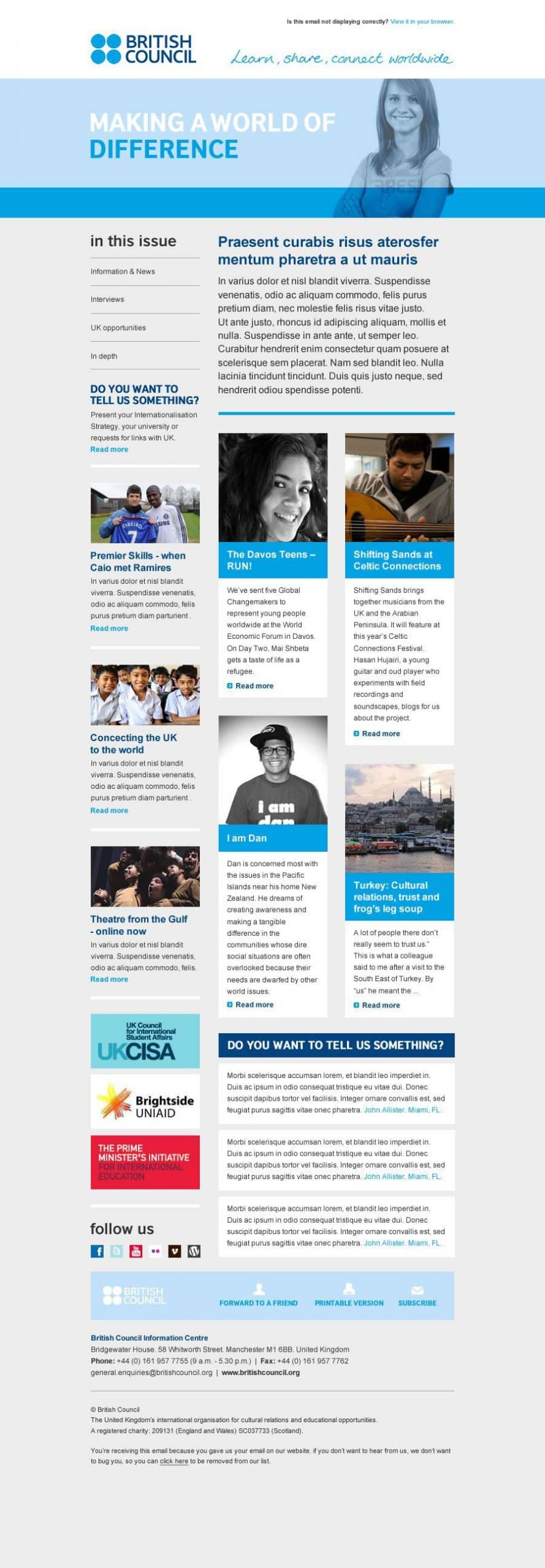Caption: 

A meticulously designed magazine layout featuring a woman prominently displayed above the caption "British Council: Making a World of Difference." The cover consists of a light blue header accentuated with dark blue trimmings, set against a sleek gray background. This issue highlights diverse stories and articles:

- The first article features a photograph of two men, likely teammates, dressed in distinct jerseys, possibly representing different sports.
- Another article showcases a smiling woman.
- A separate piece includes an image of a man playing the guitar.
- There's also an article with a photograph of four children in uniform, presumably taken at school.
- Additionally, an image features a man in a fitted cap and t-shirt, alongside a panoramic view of a city.
  
The bottom of the cover offers further information, completing this comprehensive and engaging magazine edition.